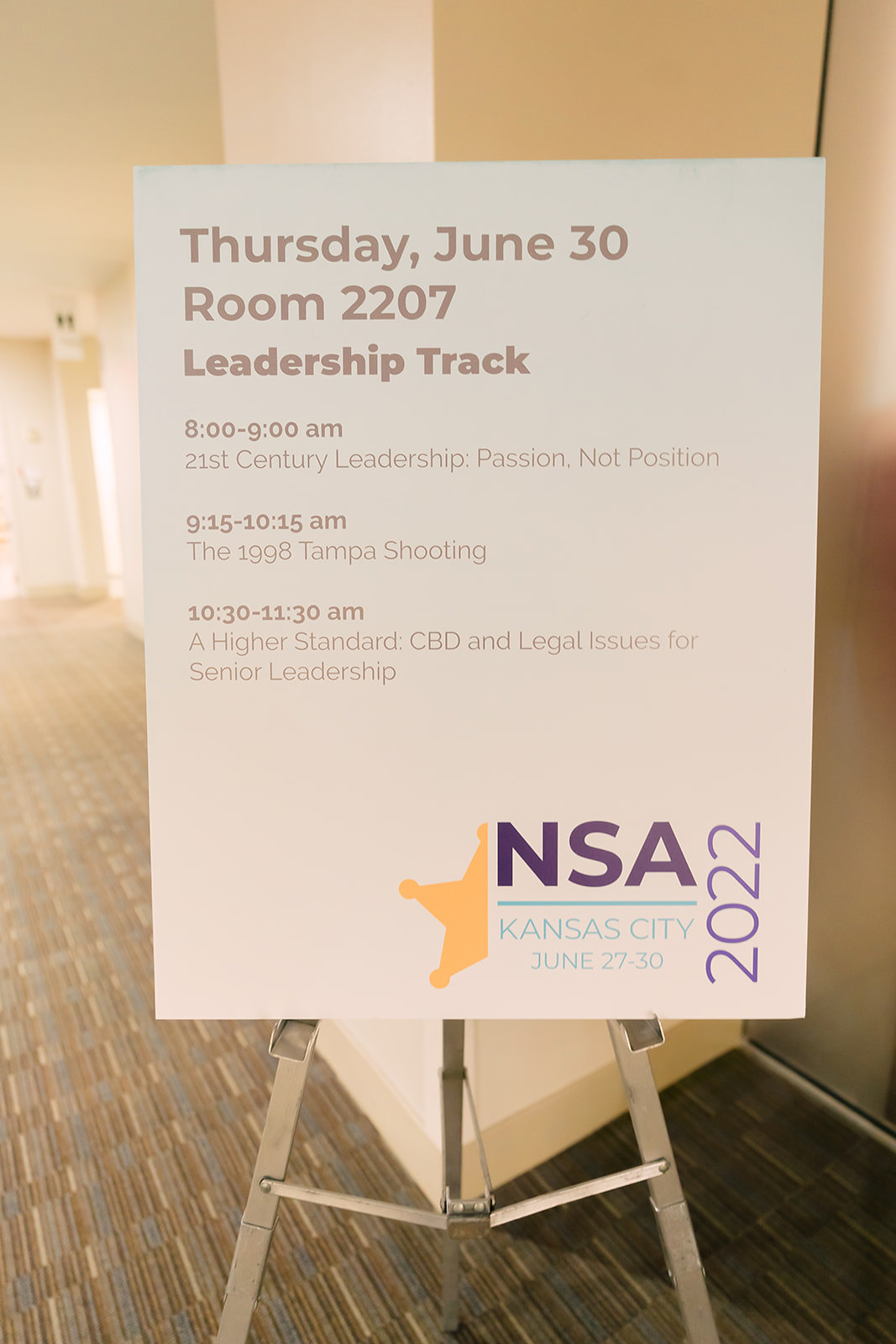This photo captures the interior of what appears to be a hallway or lobby near office spaces, perhaps in a conference venue or hotel, featuring beige walls and a brown carpet with a gray pattern. Centered in the image is a white sign with grayish-black text, mounted on a steel-colored tripod easel. The sign displays a detailed schedule for a leadership track on Thursday, June 30, in room 2207. The scheduled sessions are as follows: 8:00 to 9:00 a.m. – "21st Century Leadership: Passion, Not Position"; 9:15 to 10:15 a.m. – "The 1998 Tampa Shooting"; and 10:30 to 11:30 a.m. – "A Higher Standard: CBD and Legal Issues for Senior Leadership." The bottom right corner of the sign features a logo for NSA Kansas City, marked with a half-yellow star, indicating the conference dates of June 27 to 30, 2022.